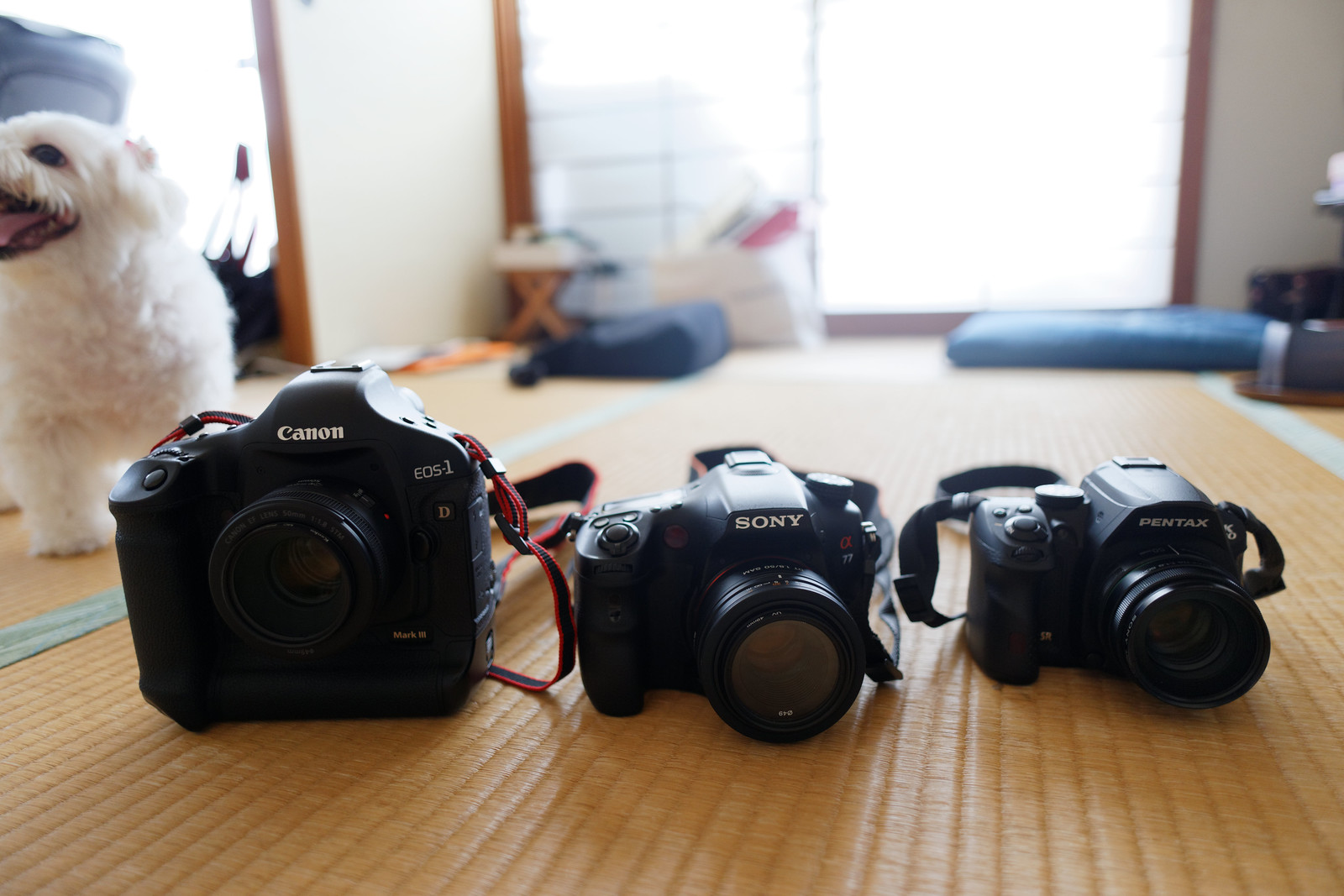In this picture, we see a trio of single-lens reflex cameras arranged on a beige wooden floor, which may have a thin bamboo mat texture. From left to right, the cameras are a Canon with an additional battery pack that makes it appear taller, a Sony, and a Pentax. These black cameras feature their straps still attached and are placed prominently in the middle of the image. To the left of the Canon is a small white dog, standing still with a happy smile, although part of its eye and mouth are slightly out of frame. The background reveals a sunny day with a large, open window flooding the room with light, partially obscuring gray lines on one side and piles of miscellaneous items in the back corners.